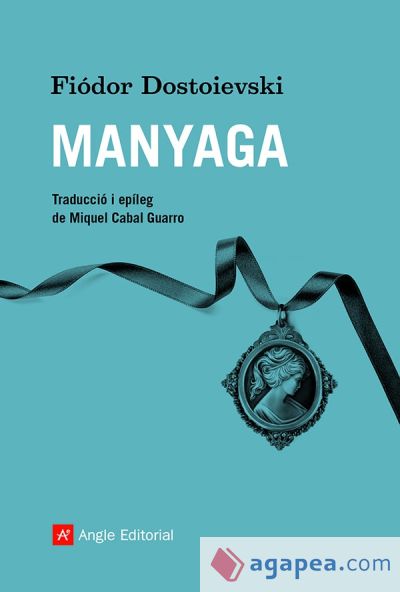The image is a rectangular mock-up of a book cover set against a Tiffany blue background. Dominating the center is a ribbon-like design in blacks and grays, with a cameo charm of an old-fashioned woman hanging off of it. At the top, black text spells out "F-I-O-D-O-R D-O-S-T-O-I-E-V-S-K-I" followed by "M-A-N-Y-A-G-A" in bold white letters. Beneath this are two lines of smaller black text in another language, mentioning "Traduccio y Epileg de Miguel Cabalguaro." At the bottom left there's a red box with a white 'A' indicating "Angel Editorial." In the lower right corner, a rectangle featuring a book graphic and the website "Agapea.com" appears in blue.